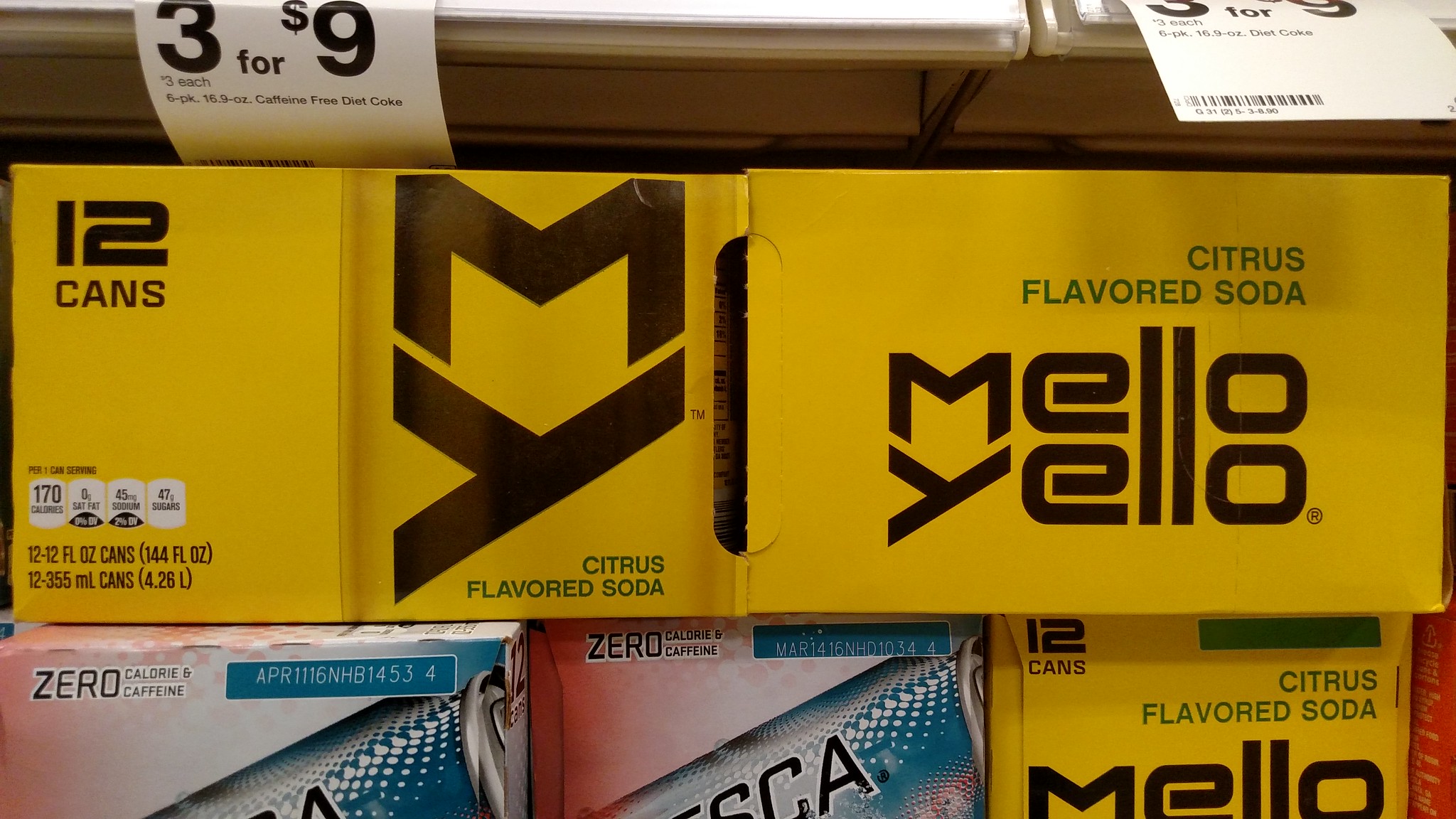This photograph showcases a grocery store shelf stocked with soda. The focal point is a yellow 12-pack of Mellow Yellow soda, which lies horizontally across two vertically stacked 12-packs of Fresca and another 12-pack of Mellow Yellow. The Mellow Yellow packaging prominently features a large "MY" in black lettering, along with the words "citrus flavored soda" in green both above and below the logo. The top left corner of the box is labeled with "12 cans" in black. Overhead, the metal store shelves partially come into view, adorned with two white price tags, each stating "three for nine dollars" with accompanying barcodes.